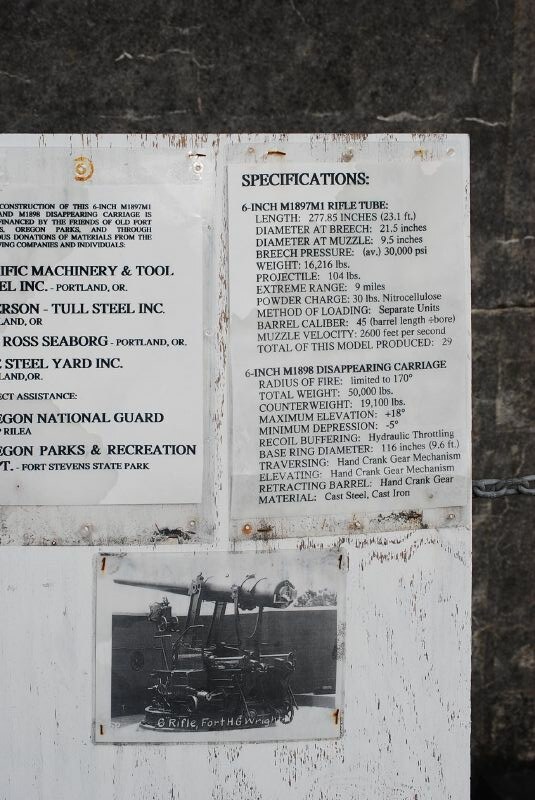The image depicts a black and white photograph of a weathered, painted white board mounted against a dark, black marble background. The board features multiple pieces of paperwork tacked or nailed onto it. Dominating the right side of the board are two detailed columns of text under headings about "specifications." The upper right section lists exhaustive details on a "6-Inch M1897 M1 Rifle 2," including specifics on its firing rate, weight, counterweights, and recoil. Below this, another column provides similar intricate specifications for a "6-Inch M1898 Disappearing Carriage." 

Prominently placed in the center below the text columns is a black and white photograph of an old cannon, labeled as a "rifle," showcasing heavy machinery held between metal supports and mounted on a large swiveling carriage. On the left side of the board, various truncated or partially obscured texts include references to "Machinery and Tool," "Portland, Oregon," "Telsteel, Inc.," "National Guard," and "Parks and Recreation." The bottom-most text appears to mention "Port Stephens State Park" along with other cut-off or slightly blurry entries. Overall, the image serves as a historical document detailing the construction and specifications of vintage military artillery from Oregon.